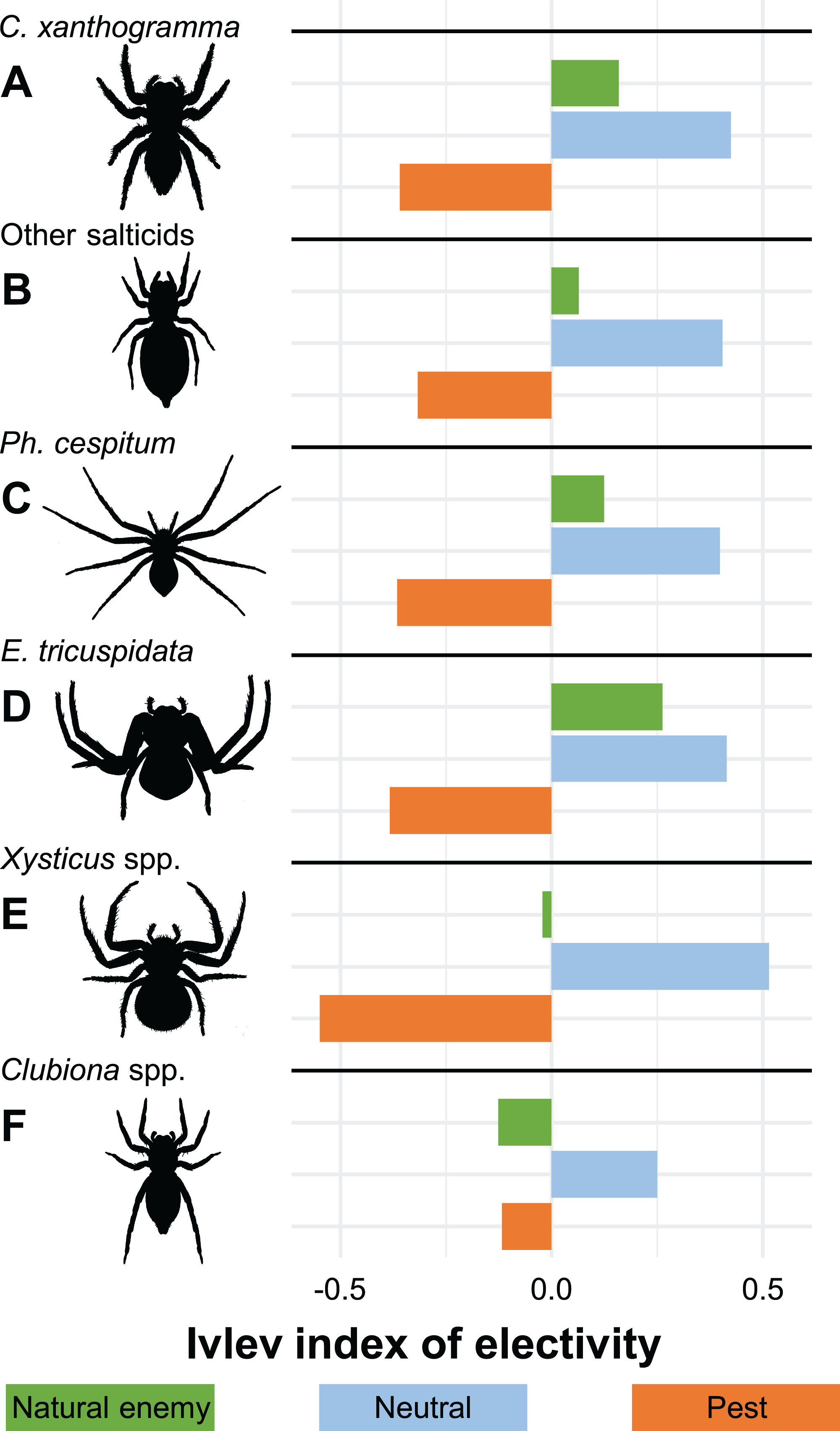The image depicts a detailed chart featuring six types of spiders labeled A, B, C, D, E, and F, with each species illustrated in black and white. Over each spider's image, its scientific name is displayed, though the names are complex and challenging to pronounce. To the right of these spider illustrations is a bar graph measured across three categories: natural enemy (green), neutral (blue), and pest (orange), based on their IVLEV index of electivity. The green bars indicating 'natural enemy' predominate the right side of the chart, while the orange 'pest' ratings are mostly on the left, except for the final spider category. At the bottom of the chart, an explanation of the color key is provided, clarifying the meanings of the green, blue, and orange bars.